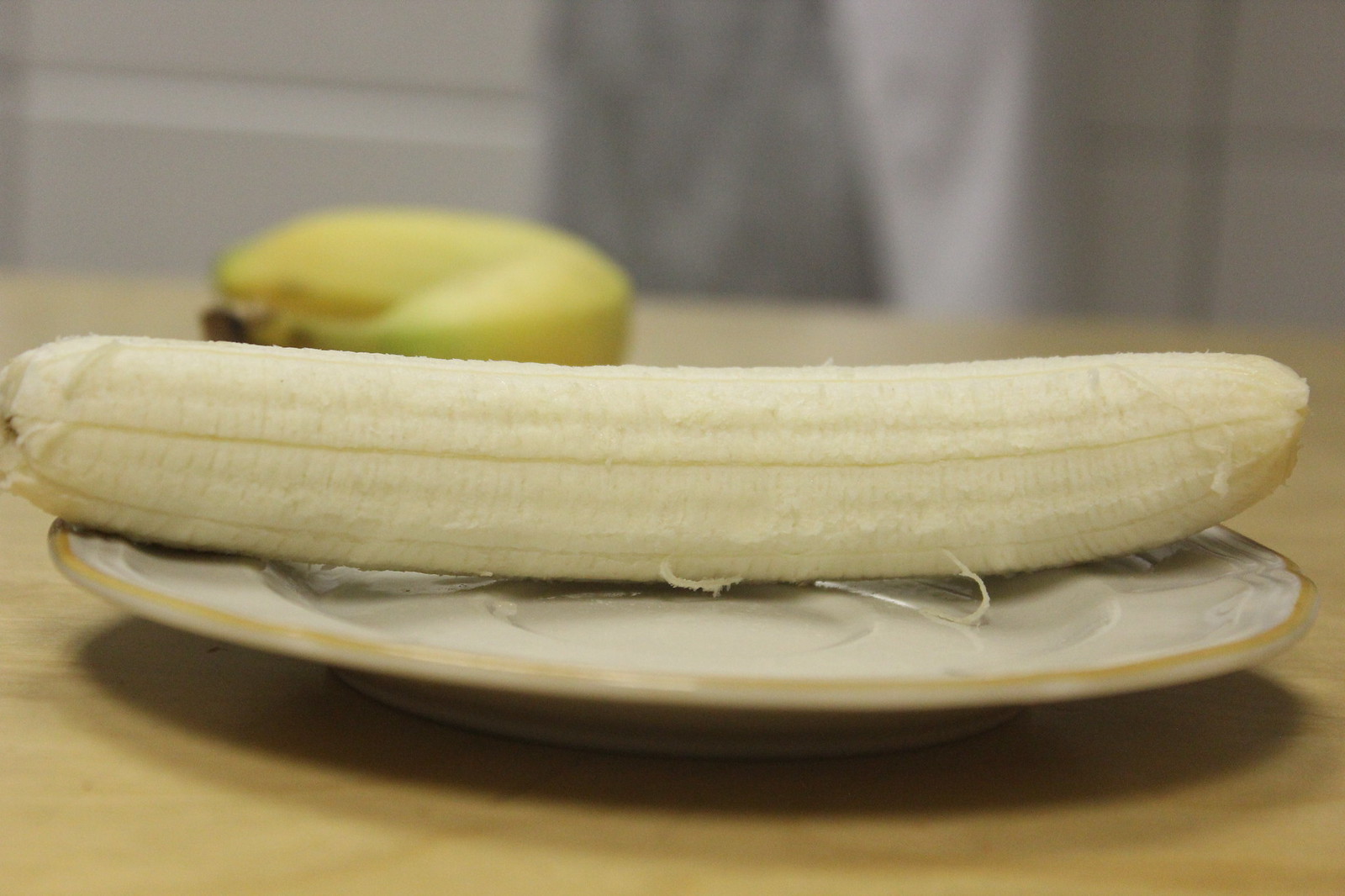In this photograph, a perfectly ripe, peeled banana is prominently displayed, resting on an elegant, light brown tan plate featuring a deep brown, textured edging. The banana still has several of the peel's inner strings clinging to its surface, adding to the natural feel of the scene. The plate, which appears to have a recessed center likely designed for a coffee or tea cup, sits atop a brown surface with a subtle wood grain, suggesting it could be a kitchen counter, island, or table. The background of the image includes an out-of-focus second banana, further adding to the casual and inviting atmosphere. Additionally, the top portion of the image is filled with light gray or medium gray vertical blurs, hinting at either drapes or possibly a person’s form near the table, contributing to the overall homely ambiance.